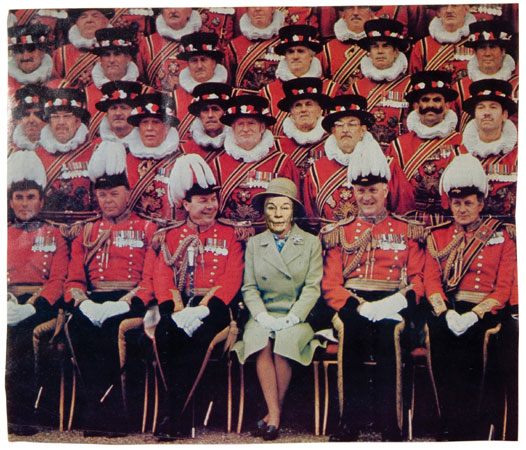The image is a square photograph depicting a meticulously arranged group of British military men and an older woman who appears to be Queen Elizabeth, though her face looks awkwardly superimposed, possibly due to lighting. The men, adorned in red uniforms with black pants, gold pinstriping, and various medals on their left chests, flank the Queen, who is dressed in a light green overcoat and short skirt with a matching short-brimmed hat. They all wear decorative hats; some with long strips of white fluff and others with brimmed designs, black rims, and red undersides. Their uniforms feature braided cords on the right chest and padded shoulders. Behind this front row, several older men in similar red uniforms with thick white collars around their necks and black top hats adorned with red, white, and black decorations form additional rows. The backdrop and composition suggest a formal royal assembly, possibly a parade, with a mix of smiles and serious expressions, capturing a distinctly British ceremonial atmosphere.